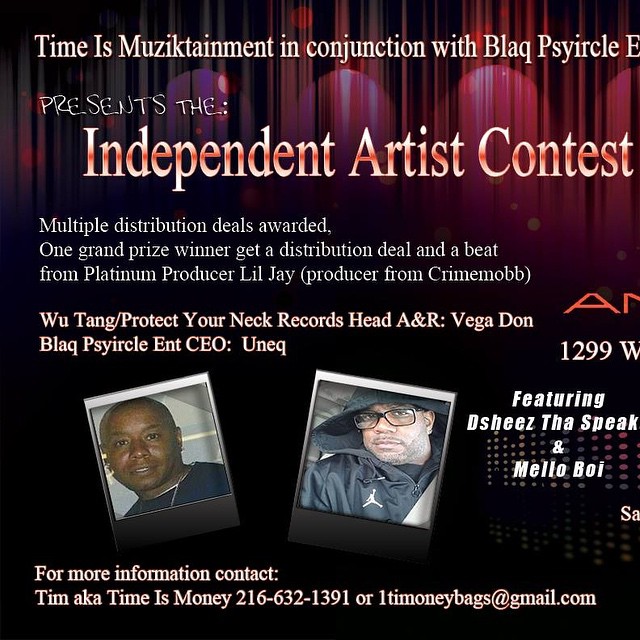The image is an advertisement for the "Independent Artist Contest" organized by Music Tainment in conjunction with Black Side Recall. The text at the top reads: "Music Tainment in conjunction with Black Side Recall presents the Independent Artist Contest. Multiple distribution deals awarded. One grand prize winner gets a distribution deal and a beat from platinum producer Lil J, producer from Crime Mob, Wu-Tang/Protect Ya Neck Records. Head A&R Bigger Don, Black Circle CEO Uneck."

The advertisement features photographs of Bigger Don and Uneck on the left side. It also mentions guest features by The Sheets That Speak and Mellow Boy. Below these images, it says: "For more information, contact Time Is Money," and provides a phone number and email for contact. The entire text is set against a black backdrop with a red curtain render above, giving it an artistic and formal look.